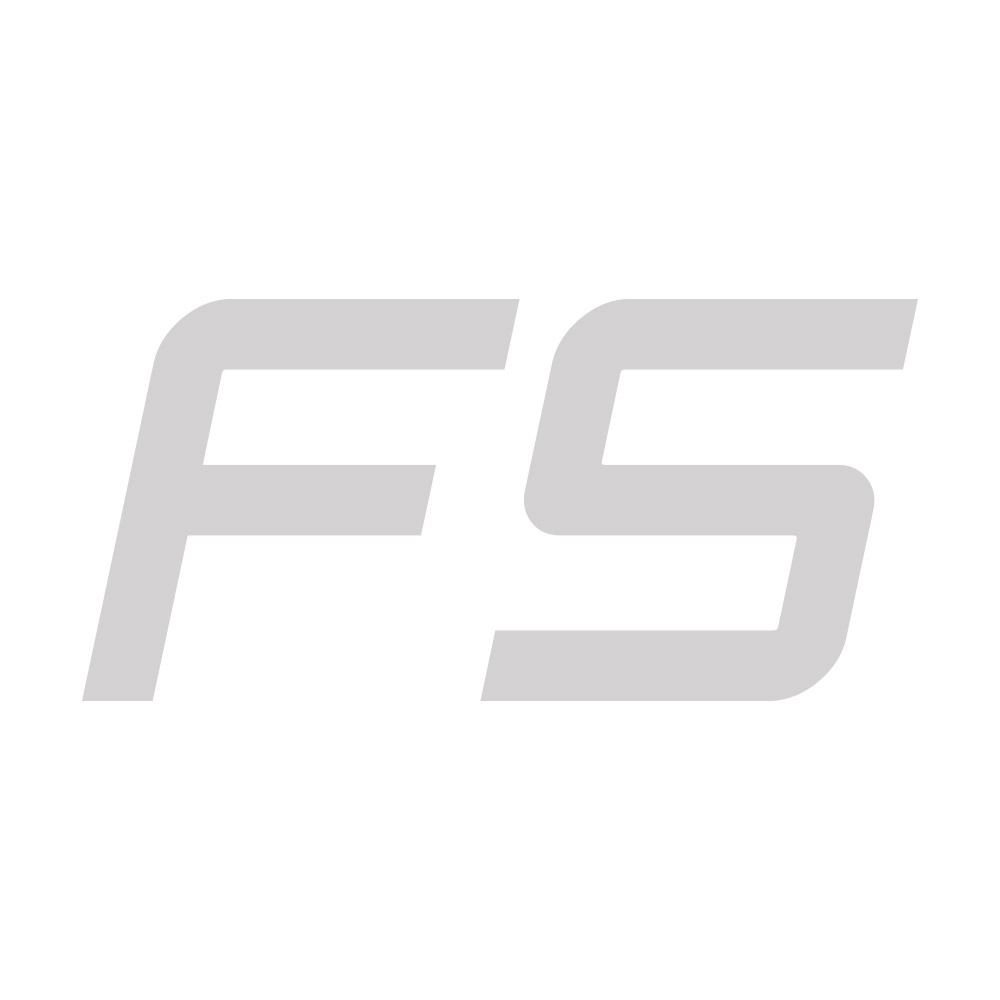The image features two very large capital letters against a solid white background. The first letter is a capital F, and the second is either a capital S or a uniquely styled number 5, which lacks the characteristic curves of an S. Both figures are rendered in a medium gray color, contrasting sharply with the plain white backdrop. The letters dominate the space, making them the sole focal points of the image. No additional text, symbols, or visual elements are present, ensuring a clear and uncluttered composition. The image is crisp and of high quality, emphasizing the stark simplicity of the design.